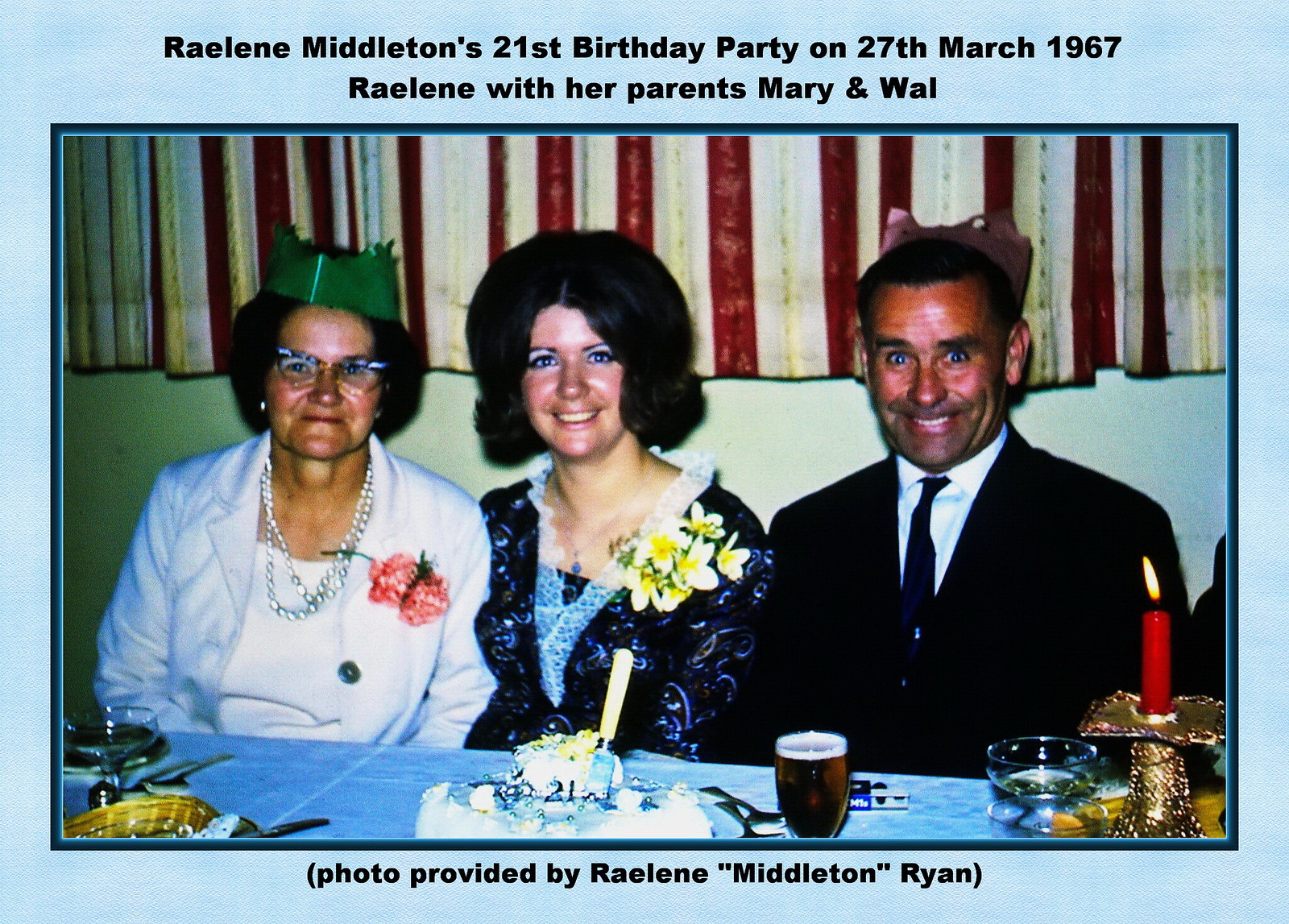This detailed image portrays Raylene Middleton's 21st birthday celebration on March 27, 1967, commemorated with her parents, Mary and Will. The photograph comes with a light blue border, framed by a red and white striped fabric backdrop. The top part of the image is captioned in black font stating the occasion and date, reading, "Raylene Middleton's 21st birthday party on 27th March 1967. Raylene with her parents, Mary and Will." Additionally, at the bottom, it mentions, "photo provided by Raylene Middleton Ryan" in the same black font.

Three individuals are seated at a table with a light blue tablecloth. On the left, Mary, an older white woman with short black hair and cat-eye glasses, is adorned with a green crown. She wears a white jacket over a white blouse, complemented by a silver pearl necklace and a pink rose corsage pinned to her left chest. Centered in the image is Raylene, a young white woman with dark, puffy hair. She is dressed in a blue and white lace ruffled dress, accentuated by a yellow corsage on her left. To the right, Will, a white man with dark hair and striking blue eyes, wears a black suit with a dark tie and a white shirt.

On the table in front of them, there are drinking glasses, candles, and a cake with the number "21" visible, along with a knife, indicating the celebratory nature of the scene. A cup of champagne is also present, adding to the festive atmosphere. The intricate details and arrangement nicely highlight the historic and joyous moment of Raylene's milestone birthday with her family.